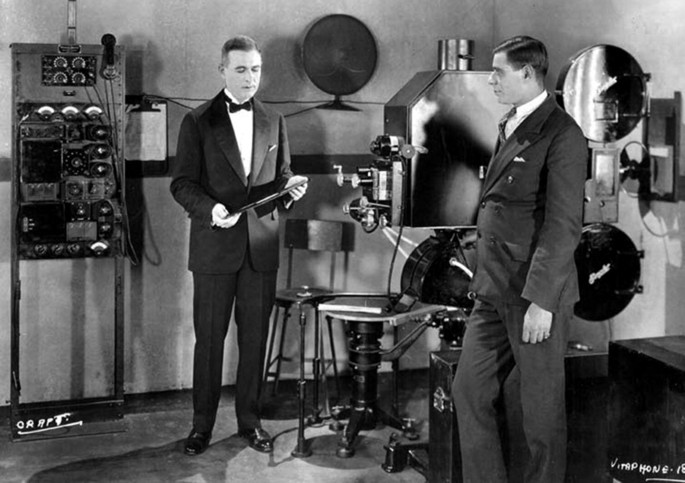In this early 20th-century black and white photograph, likely taken in the 1920s, we observe two middle-aged gentlemen engaged in conversation, set in a well-lit, industrial-looking room. This promotional photograph, released by Western Electric (a precursor to AT&T) or Bell Labs, features their Vitaphone film sound system, pivotal in the advent of sound in motion pictures around 1926. 

To the left, one man, clean-shaven with short hair and dressed in a dark suit complemented by a bow tie, holds an electrical apparatus, explaining its function. To his right, slightly closer to the camera, another man, also clean-shaven and with short hair, listens intently. He is dressed in a lighter-colored suit, still dark, paired with a white shirt and tie.

Behind them, a variety of early 20th-century electrical and motion picture equipment fills the room. An imposing piece of machinery, likely a motion picture projector with a lens and two film reels stacked vertically, dominates one side. Nearby, an electrical board with numerous dials, buttons, and wiring stands against the wall. Additionally, a speaker appears to hang from the wall, while a stool sits amid the scattered instrumentation.

This detailed scene, capturing a pivotal moment in cinematic history, underscores the technical advances of the time, heralding the era of "talkies" in film.